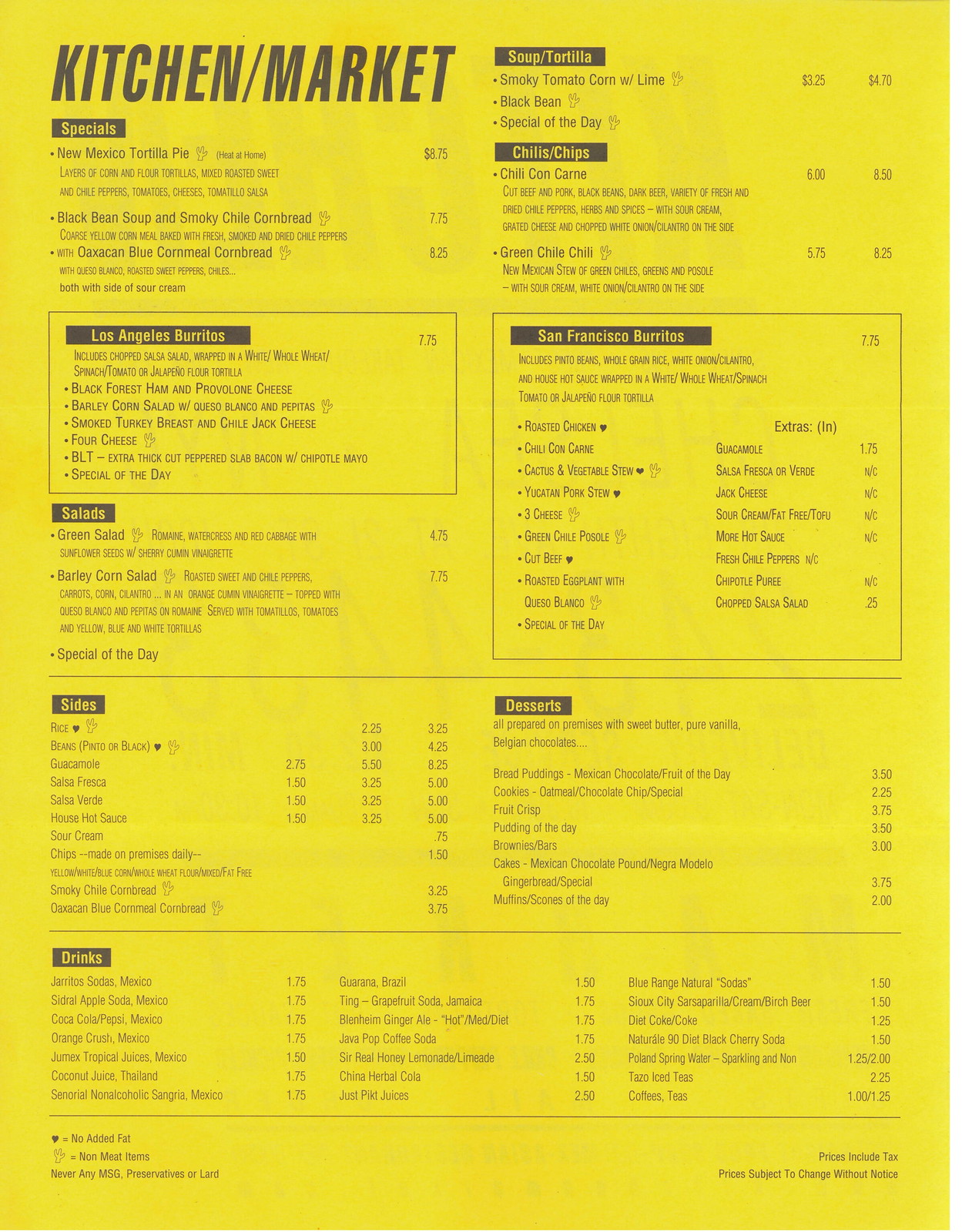The image showcases a vertically oriented rectangular menu against a bright, sunny yellow background with no discernable texture. Subtle shadows are cast on the menu, creating slight variations in tone, primarily due to lighting effects. The menu itself is printed in stark black text on a transparent surface, allowing the black writing to be visible from the other side.

At the top, the menu prominently features "KITCHEN MARKET" in bold, uppercase black letters. Below this, a small black rectangle with the word "SPECIALS" in white text separates the header from the main content. The menu is organized into various sections detailing different offerings:

- **Kitchen Market**: At the top, with bold, uppercase black letters.
- **Specials**: A section highlighted in a small black rectangle with white text.
- **Los Angeles Burritos**: Listed within a black-outlined rectangle with a small black header showing the title in white text.
- **Salads, Sides, Drinks**: Following in the left column.
- **Soup/Tortilla, Chili/Chips**: Listed in the right column.
- **San Francisco Burritos**: Another black-outlined rectangle with a white-titled black header.
- **Desserts**: Below the burritos listing.

Towards the bottom, the menu includes a legend explaining symbols used to denote items with "no added fat," "non-meat," and "no MSG, preservatives, or lard." An additional note clarifies that prices include tax and are subject to change without notice.

This detailed depiction of the menu offers an organized layout and clear categorizations, serving as an informative guide to potential diners.